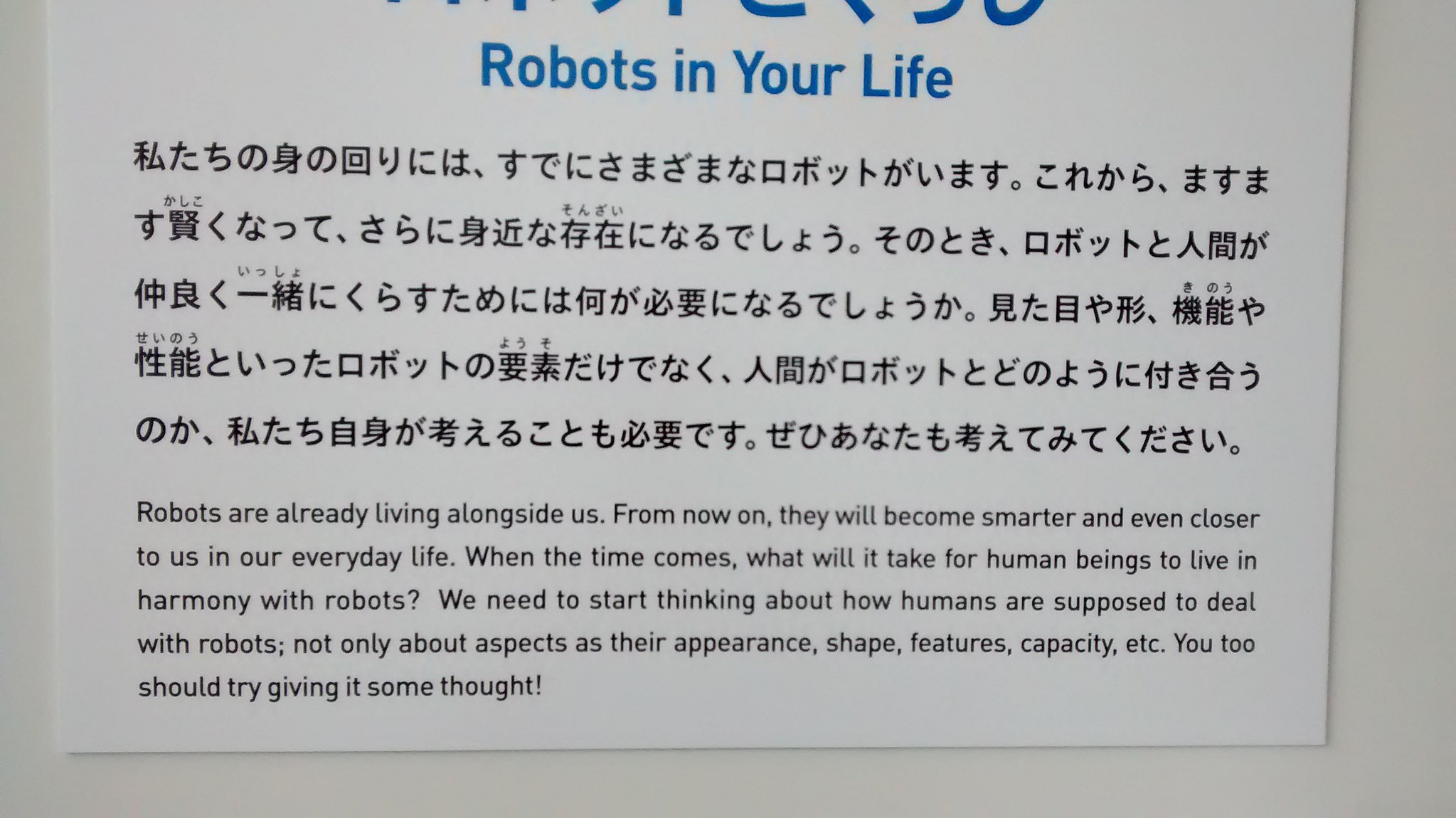The image features a predominantly white sign posted on an off-white wall, occupying most of the frame. At the very top of the sign, the heading "Robots in Your Life" is written in blue font. Below this heading, there are five lines of text in what appear to be characters reminiscent of Chinese or Japanese, though their exact nature is unclear. The text in these characters is followed by a translated message in small black font. The English text reads: "Robots are already living alongside us. From now on, they will become smarter and even closer to us in our everyday life. When the time comes, what will it take for human beings to live in harmony with robots? We need to start thinking about how humans are supposed to deal with robots, not only about aspects as their appearance, shape, features, capacity, etc. You, too, should try giving it some thought."